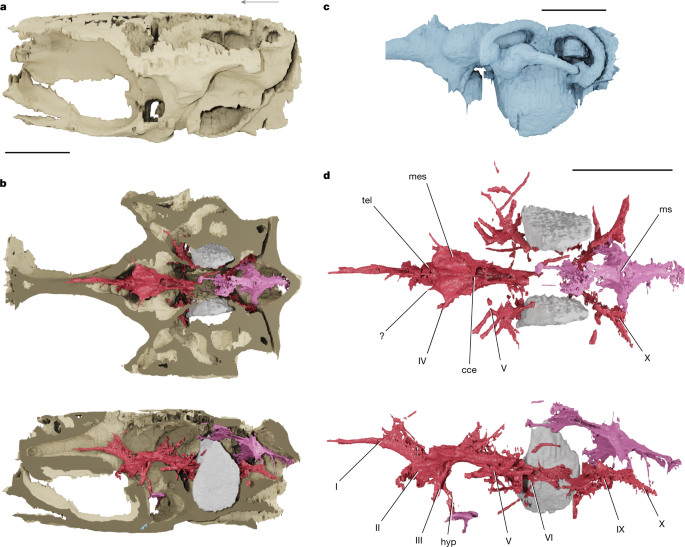This image is a detailed 3D rendering consisting of six sections, labeled A, B, C, and D at the top and two additional unlabeled sections at the bottom. The overall theme appears to be anatomical, perhaps focusing on a skull and the interior of a brain or other internal structures, possibly from an animal resembling a dog.

- **Section A** (top left) is depicted in beige and tan tones, resembling an oval shell or exoskeleton with a large hole at its center, suggestive of a skull with an open jaw. 
- **Section B** (directly below A) is similarly beige and taupe but includes a pink interior, potentially depicting a cross section of internal organs or skeletal structures. This section evokes the appearance of a man-of-war or fish cross-section, highlighting a mix of beige exterior and pink internal components.
- **Section C** (top right) displays in a bluish-gray hue, with a misshapen, organ-like structure. It lacks detailed textual labels beyond generic annotations such as "TE," "MES," and a question mark indicating points of interest without clear identification.
- **Section D** (directly below C) is another irregularly shaped object with multiple annotations pointing at its interior, with labels such as "Question Mark," "Numeric 5," "CCE," "Numeric 3," and "X." This section may portray complex internal components.
- The two lower, unlabeled sections provide further intricate cross-sections or different views of what appears to be the same anatomy shown above, displaying a mix of grey, red, and purple tones representing various internal structures, potentially surrounding or including parts of the brain.

Overall, the image constructs a complex anatomical study with detailed visual layers, lacking explicit textual explanations but offering a profound exploration of the internal structure, possibly prepared for pre-surgical analysis or academic study.